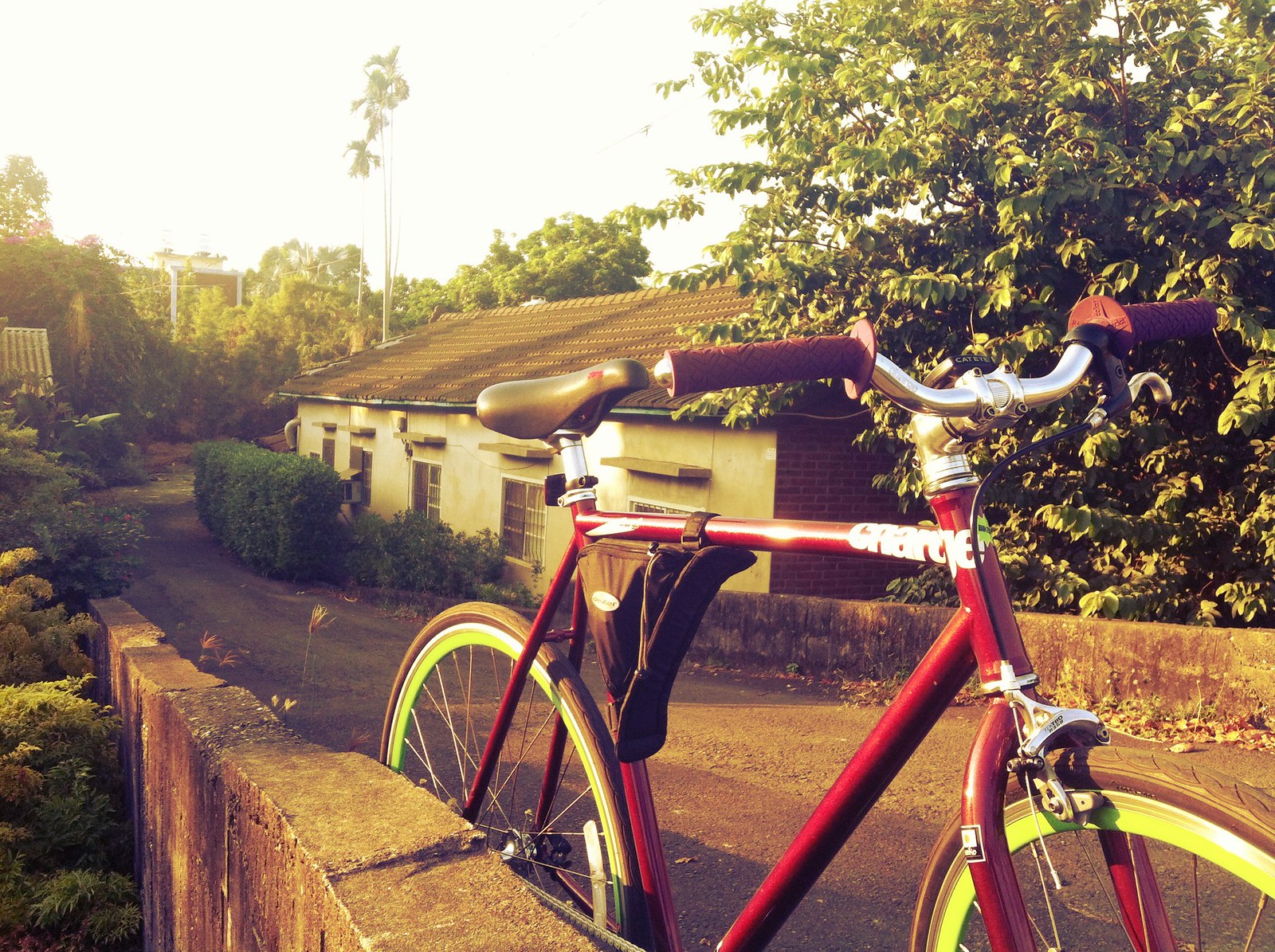The photograph captures a striking, vintage-like scene featuring a dark red road bike with neon fluorescent yellow wheels, standing on a wide cement pathway that appears to be part of a bridge or roadway flanked by cement walls. The bike, positioned in the bottom right quadrant of the image, faces right with its handlebars, while its back wheel points left. It boasts a black seat and red handlebars, with a triangular-shaped bag nestled in its frame. Dominating the background is a single-story building constructed with brick and plaster, showcasing a tiled roof and five visible windows, around which the road curves. Surrounding the scene are lush, green trees and bushes, under a sky that is bright yet greyish-yellow, suggesting the sun is high but diffused.